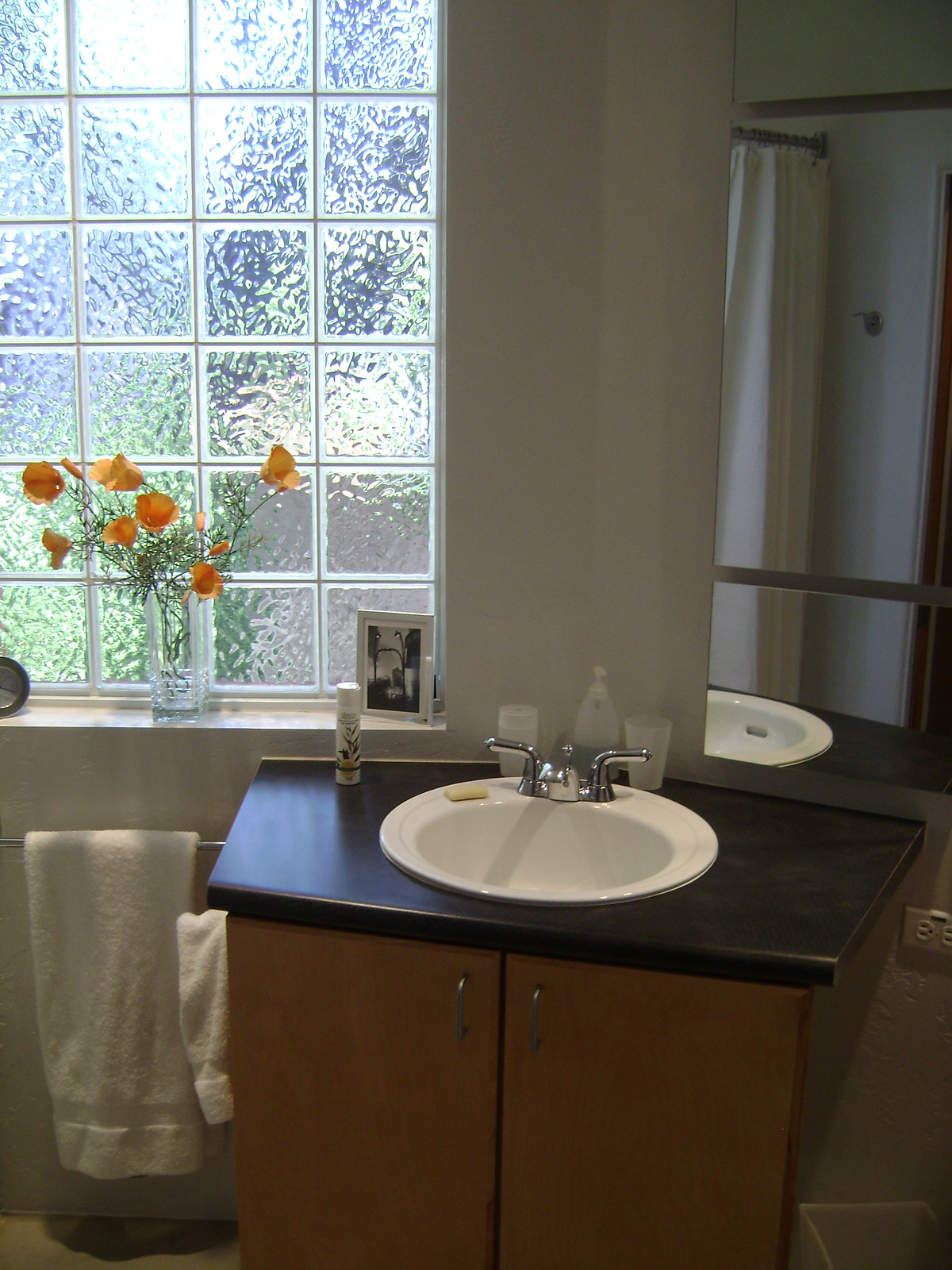The image depicts a modern bathroom scene. On the left side, there is a frosted glass window divided into a grid of small squares, offering a blurred view of green, white, and blue hues outside. Adorning the windowsill is a glass vase filled with vibrant orange flowers, accompanied by a small white picture frame that contains a black-and-white photo, the details of which are indistinct. Below the windowsill is a wall-mounted towel holder with a neatly draped white towel.

Adjacent to the towel holder is a sleek vanity unit, featuring a black countertop and a white sink embellished with silver hardware. The vanity has brown cabinet doors, accented with silver handles, and a small hand towel hangs off its side. A mirror mounted on the wall above the vanity reflects part of the bathroom, including the shower curtain and the sink, adding depth to the scene.